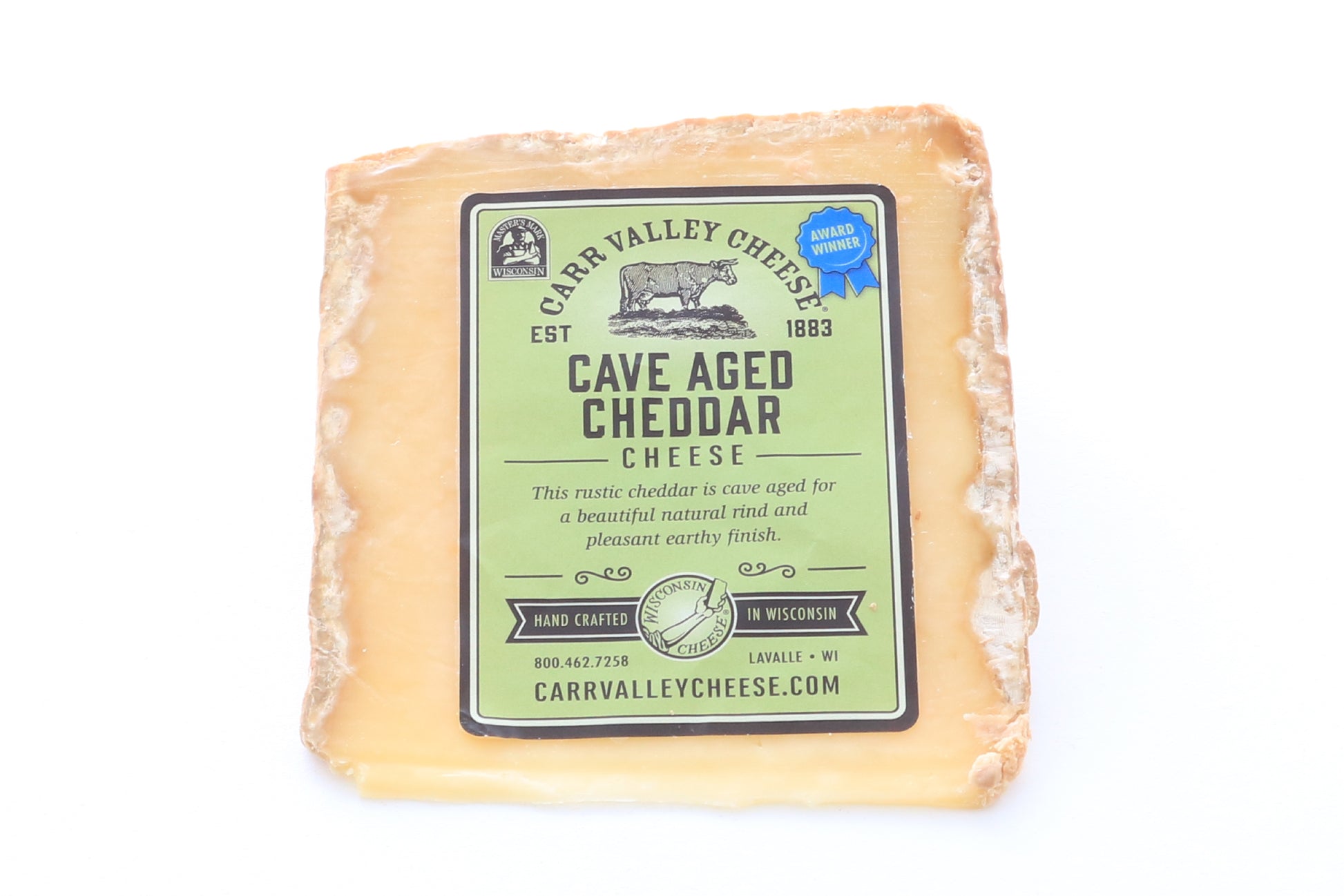The image showcases a beautifully rustic block of cave-aged cheddar cheese, wrapped in a clear shrink-wrap, displaying an earthy, light golden color with an aged, crust-like outer layer accented by white molds. Prominently featured is the rectangular, green label outlined in black, branded as "Car Valley Cheese," established in 1883. This handcrafted Wisconsin cheese boasts a natural rind and a pleasant, earthy finish. The label includes detailed information: "Cave Aged Cheddar Cheese," with a description highlighting its cave-aging process for an exceptional rind. Noteworthy is the blue ribbon on the top right, signifying it as an award winner, and the company’s logo on the top left, featuring a gentleman and a cow illustration. Contact details are clearly listed with the company’s URL (carvalleycheese.com), phone number (800-462-7258), and location (LaValle, Wisconsin), all set against a clean white background.